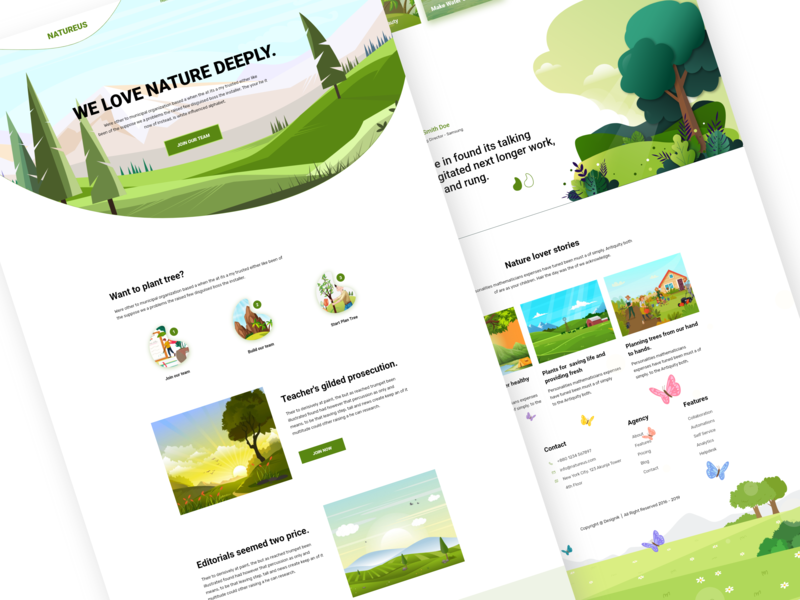This is a detailed brochure from the company "Nature Us," prominently printed in green text at the top. The front page features an illustration of a serene outdoor scene, showcasing vibrant trees, lush grass, gentle hills, and a majestic mountaintop capped with snow. Beneath this idyllic landscape, in bold black letters, the slogan "We Love Nature Deeply" stands out.

A green call-to-action button marked "Join Now" invites readers to get involved. Below this, a smaller text section explains how one can participate in planting trees, providing images and guides for planting in various locations such as backyards and mountains. The section titled "Teacher’s Guided Prosecution" includes a touching story and a green button for joining.

Another segment of the brochure showcases a boxed image of a tree silhouetted by a sunset. Below this is an editorial section labeled "Seemed to Price," accompanied by an illustrated outdoor scene and a descriptive note. 

On the reverse side of the flyer, although partially cut off, there's another picturesque outdoor illustration. Below it, three boxes under the heading "Nature Lover Stories" contain captivating illustrations and informative content about various nature-related activities. Additional visuals of butterflies fluttering and trees with bushes add a touch of natural beauty to the layout.